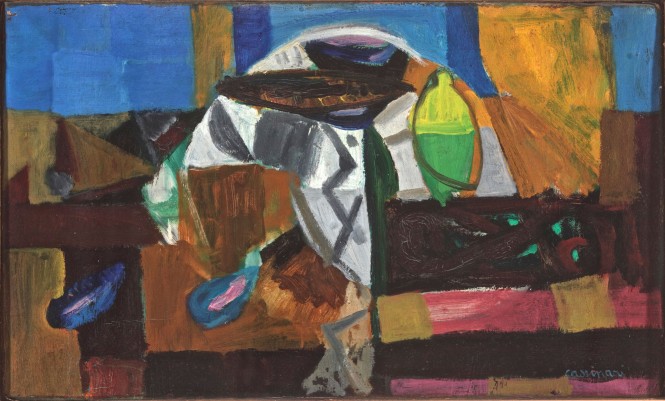The painting, seemingly acrylic, presents a stylized and abstract depiction of a bedroom. Dominated centrally by a large, tent-like white figure with gray or black striped patterns, the figure has a door-like feature. The background consists of a series of brown rectangular and square shapes, which appear less detailed, possibly serving as a backdrop. Diverse shades of blue fill the upper portion of the painting in blocky patterns, while additional pink and purple hues are scattered near the bottom right. Among these elements are two teardrop-shaped blue forms with pink ovals located towards the left of the figure. There's also a green and yellow drinking bottle positioned on a table. The artist's signature, KAMONARU, is visible at the bottom right corner of the painting.